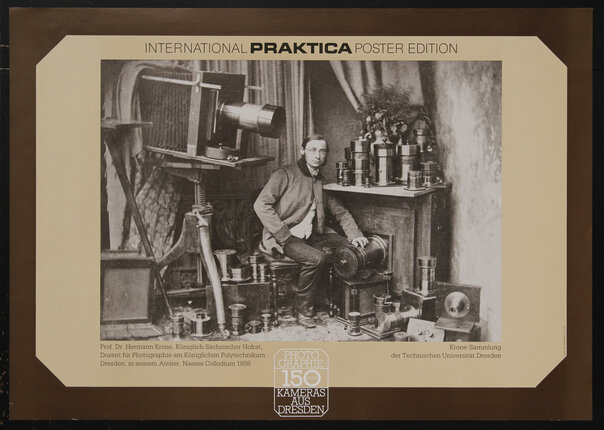Framed in a horizontally aligned rectangular picture frame with a dark brown or black border, this image is a detailed composition with a layered design. The innermost area is bordered by a thick, angled brown section that forms an eight-sided tan outline around a central black-and-white photograph. The top of the tan section prominently features "International Practica Poster Edition" in bold black letters.

The black-and-white photograph depicts a man sitting on a chair, looking towards the viewer. He wears glasses, a jacket over a white shirt, and dark pants. To his left is an old-fashioned, large camera, and to his right, his hand rests on a cylindrical metal object. Surrounding him are various pieces of camera equipment, including possible camera lenses on shelves directly above him.

At the bottom of the photograph, centered in white text on a white box, it reads "Photography 150 Kammerer’s Ost Dresden." There is also finer, smaller black text visible in the lower left and right corners, although the exact wording is not entirely clear due to its small size. This image captures a historical depiction of a man amidst an array of vintage photographic equipment.